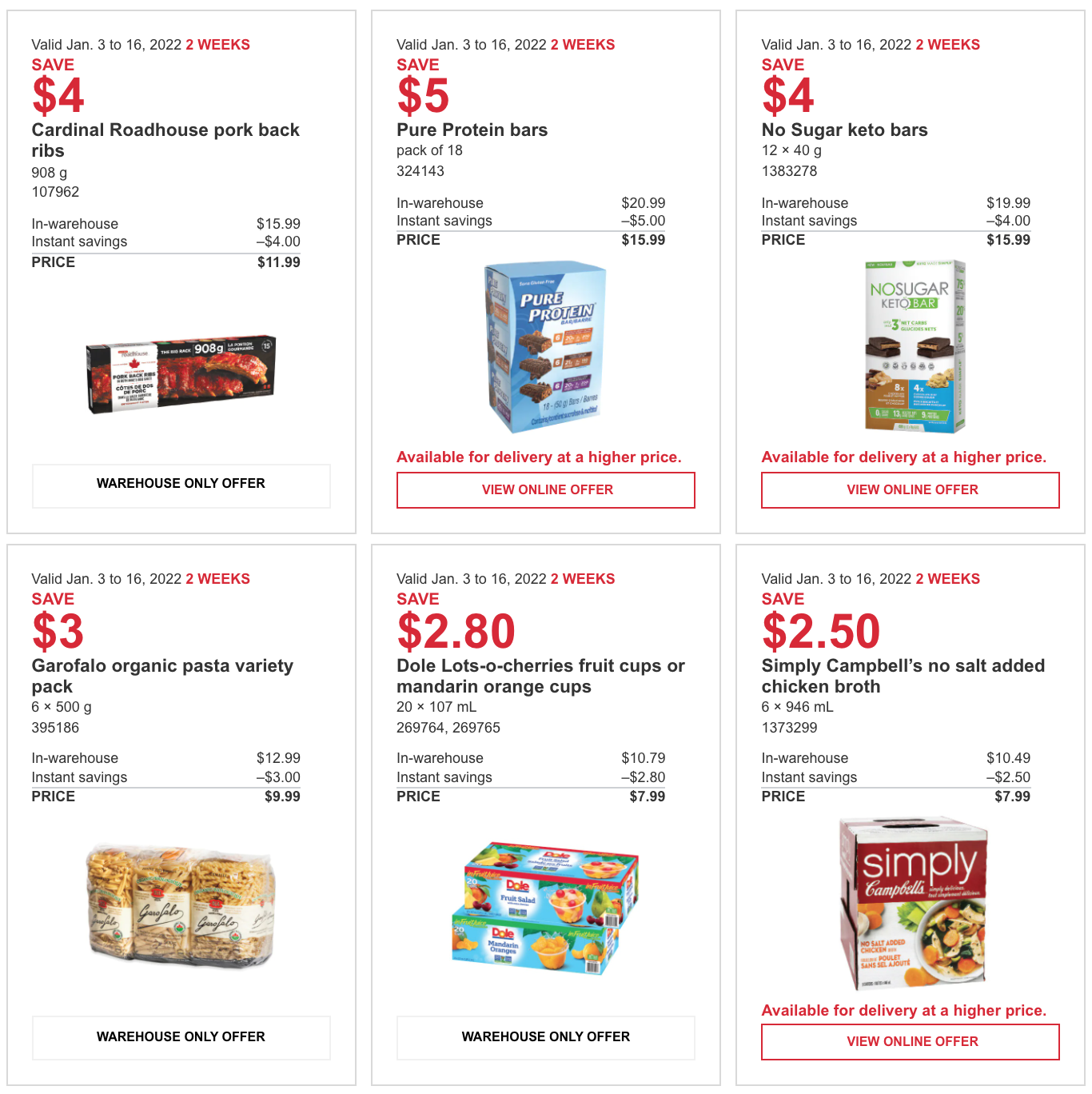This image is a screenshot showcasing six different deals from an unspecified website. The offers are divided into two categories: 'Warehouse Only' and 'Online Offers,' with three deals in each category. All six offers are valid from January 3rd to January 16th, 2022. At the top left-hand corner of each deal, the text "Two Weeks Only" is prominently displayed in bold red font.

For each offer, the discount amount is highlighted in bold red font just below the validity period, indicating savings such as "$4 off" or other specified amounts. The product name follows in bold black font, with the product quantity or weight listed underneath. An item number is provided below the quantity/weight for further identification.

The pricing structure consists of several key details:
- The warehouse price is shown, followed by the instant savings amount.
- The final price, after the discount, is prominently displayed in bold black font to the far right.

Each offer includes an image of the product, ensuring easy recognition whether you are shopping in-store or online. For products available online, a red-outlined box with bold red font indicates "View Online Offer," and above this box, the text "Available for delivery at a higher price" clarifies the terms, eliminating any confusion.

In summary, this screenshot illustrates three 'Warehouse Only' deals and three 'Online Offers,' each clearly marked with validity dates, discount amounts, product details, and final pricing, all supported by corresponding product images.